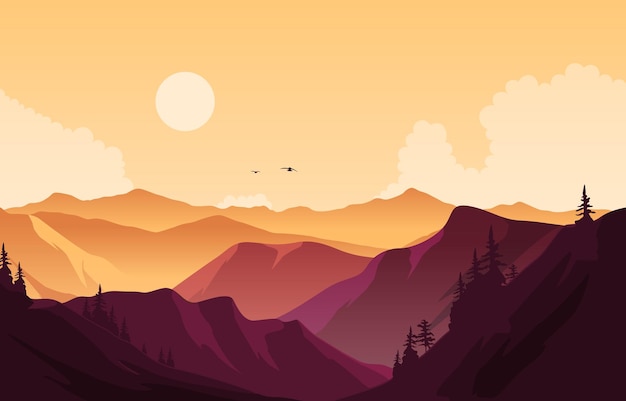This AI-generated 3D landscape image features an intricate, multi-layered mountain range extending into the distance. The sky, tinted a tan color transitioning to light beige clouds, serves as the backdrop. At the horizon, the steep, prominent mountains are golden, giving way to pink and purple mountains as they move closer to the viewer. Two mountains on either side are shaded in lighter purples, while the nearest mountains are darker purple and adorned with silhouetted trees. A bright moon hangs in the sky, accompanied by two birds, possibly geese, flying in graceful arcs. The landscape features a series of peaks and valleys, with the mountains blending from a yellowish-orange hue in the background to more violet-pink hues in the foreground. The overall scene is bathed in warm, glowing light, enhancing the vivid contrast between the different colors and layers of the mountains.